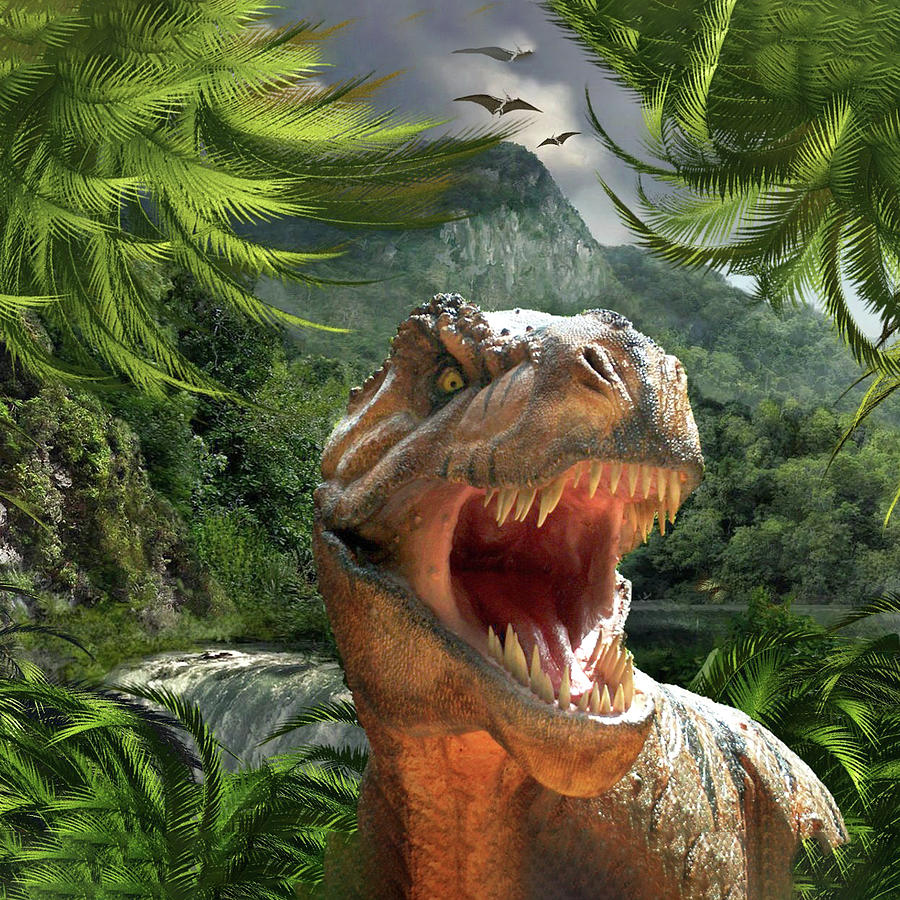This digitally rendered image portrays a lifelike Tyrannosaurus rex in vivid detail, captured in a dramatic, ferocious pose. The T-Rex dominates the foreground, facing forward with its mouth wide open, revealing its sharp teeth and deep throat. Its skin displays a mix of orange and brown hues, contributing to its menacing appearance. One eye is clearly visible on the left side of the image, adding to the realism. Surrounding the T-Rex are lush palm fronds, with a dense array of trees and green foliage extending into the background, alongside a serene lake and a cascading waterfall. The scene is set against mountains draped in verdant trees, while the sky above is filled with gray clouds and several flying dinosaurs, reminiscent of pterodactyls, adding to the prehistoric ambiance. This detailed and dynamic scene looks like it could belong in a movie such as Jurassic Park or a theme park exhibit, yet seamlessly blends elements of digital artistry and natural wonder.